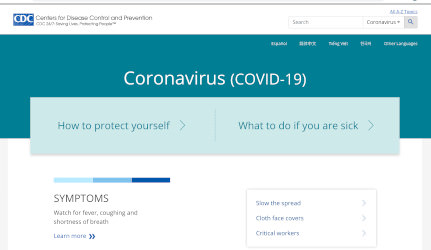This image is a screenshot of a webpage from the Centers for Disease Control and Prevention (CDC) concerning the coronavirus. At the top left corner, the CDC’s logo is visible, signifying that the content is authoritative. The webpage is dedicated to providing information on COVID-19, focusing on how individuals can protect themselves and what steps to take if they are infected.

The webpage has a light bluish-green background, with white text prominently displaying important information. Sections are divided by thin lines, creating a clean and organized layout. On the left side, there are several links resembling buttons, each addressing crucial aspects related to the virus.

At the bottom left of the screenshot, there's a section titled "Symptoms," which is highlighted in brown. It advises readers to watch for signs such as fever, coughing, and shortness of breath, accompanied by a "Learn More" link marked with two blue arrows pointing to the right.

On the bottom right, another section emphasizes slowing the spread of the virus, highlighting the use of cloth face covers and critical worker guidelines.

Finally, at the top right corner of the page, there's a search bar for users to look up additional information on the CDC website. Despite the screenshot being somewhat blurry and small, the layout and critical information points can be discerned.